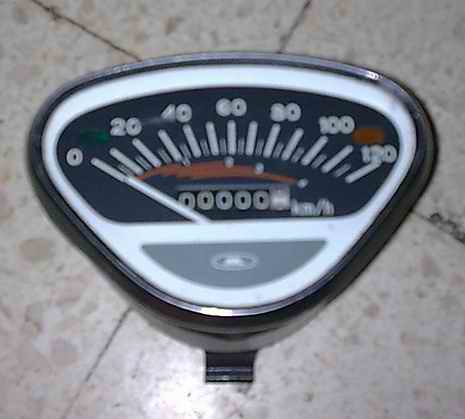The image depicts a scale used for weighing individuals, placed on a tiled floor consisting of four white tiles that intersect at the scale's location. The scale has a unique design, with its overall shape being somewhat round but tapering into a rounded triangle at the top. It features a silver, metallic outer edge and a white inner edge, giving it a stylish appearance. 

At the bottom of the scale is a gray semi-circular section that appears to contain a symbol, but due to the blurriness of the image, the details of this symbol are indiscernible. The measurement dial of the scale is marked with numbers from 0 to 120 in 20-unit increments, with smaller bars indicating 10 and 5-unit increments. These markers are highlighted in white. Notably, between the 0 and 20 marks, there's a green splotch, and between the 100 and 120 marks, there's a red splotch. Below the numerical markers is a significant, wispy red mark that adds to the visual complexity of the scale's interface.

A long, white dial points to the weight measurement, and beneath the red splotch, there are six numbers displayed, with five zeros clearly visible, and the final number appearing between values. Accompanying these numbers is an inscription that seems to include the letters "KM," although the exact characters are unclear. It’s likely that the scale measures weight in kilograms, as the maximum value is 120 kg.